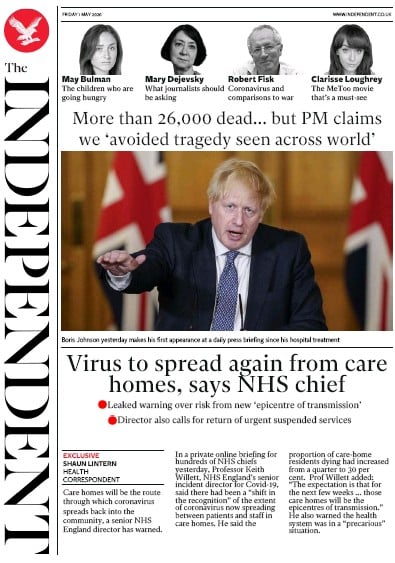Screenshot from "The Independent" showcasing a prominent news story in a vertically formatted layout.

At the center of the screenshot is an article featuring Boris Johnson, standing in front of a microphone and speaking, with UK flags prominently displayed in the background. The headline reads: "Boris Johnson makes his first appearance at a daily press briefing since his hospital treatment."

Additionally, the screenshot includes another main article titled: "Virus spread again from care homes, says NHS chief."

At the top, there are images of four editors, three women and one man, next to their respective op-ed articles. The featured editors are:
- May Bullman, with an article titled "The children who are going hungry."
- Robert Fisk, with an article discussing "Coronavirus in comparison to war."

The screenshot also displays "The Independent" logo and design elements, including a red circular outline with the words "Word of Prey." The format appears to be aligned more with mobile viewing.